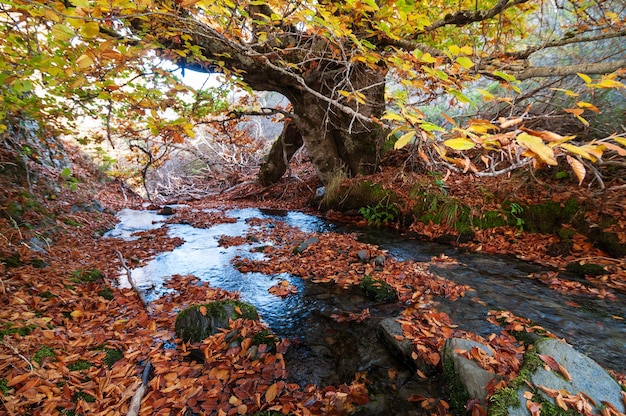This is a beautiful nature photograph capturing a serene autumn scene in the woods. The image, presumably taken in fall, features a massive, ancient tree with a thick trunk that spans at least 10 feet across. Most of the frame is dominated by this tree, which displays greenish-yellow to light green and completely yellow leaves, creating a vibrant canopy. Below the tree, a shallow creek or stream flows, bordered by a steep embankment. The stream's surface reflects the bright blue sky, although parts of the water appear very dark where shaded. The creek is scattered with reddish-orange and brown dried leaves, some stationary and some slowly drifting, creating the illusion of a still lake despite ripples indicating gentle motion. There are gray rocks with patches of moss situated to the right of the image. The overall scene is bright and vivid, showcasing the natural beauty of an autumnal woodland landscape.